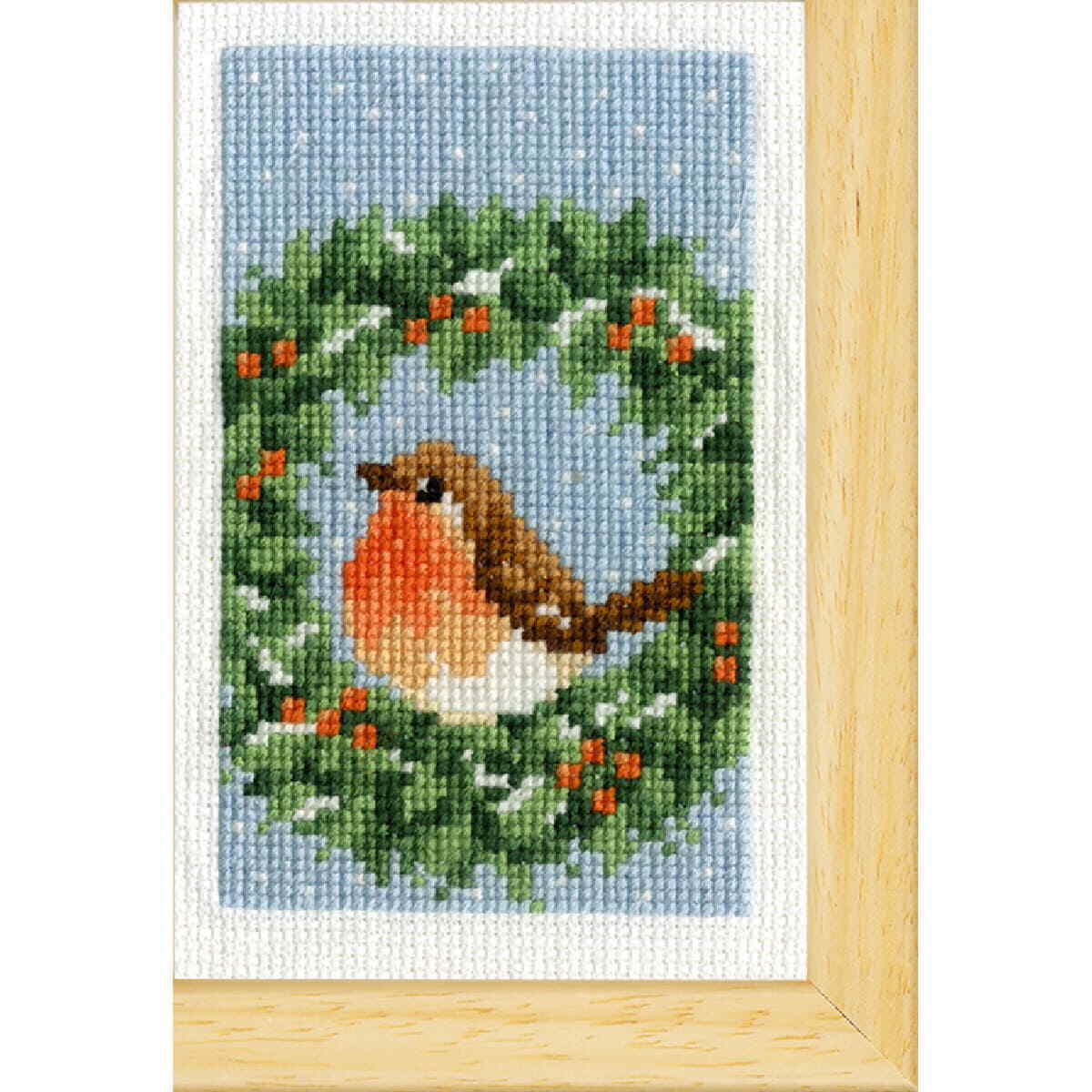This detailed image portrays a vertically aligned, rectangular finished cross-stitch artwork, framed in a light wooden frame visible on the right side and bottom edges. The cross-stitch piece features a white-bordered blue background speckled with small white flecks, evoking a snowy scene. Central to the composition is a lush, circular wreath adorned with varying shades of green and accented by red berries and small hints of white, suggesting snow. Perched in the center of the wreath is a chubby robin bird, characterized by its brown back and tail, white underside, and vivid red-orange breast. The robin's dark brown beak and beady black eyes add to its charming appearance. The intricate details and framing suggest this is a carefully completed and possibly displayed or for sale piece of cross-stitch art.